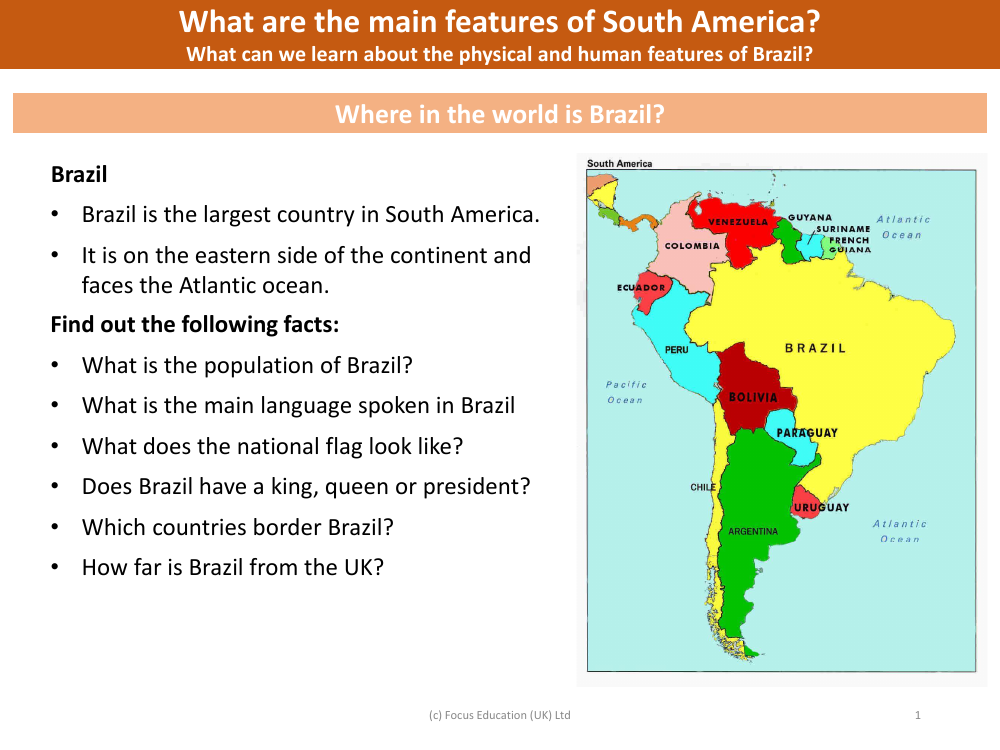The image appears to be from an educational website, possibly focused on teaching geography. At the top of the screen, a brown box contains white text asking, "What are the main features of South America?" Below this, in a smaller font, it asks, "What can we learn about the physical and human features of Brazil?"

The background of the image is predominantly white. Beneath the brown box, a peach-colored box with white text poses the question, "Where in the world is Brazil?" This section also lists some facts about Brazil in black font. To the right of these facts is an enlarged map of South America, showing Brazil prominently in yellow, with the surrounding countries in various other colors. The Atlantic and Pacific Oceans are labeled on either side of the continent.

Some of the listed facts include:
- Brazil is the largest country in South America.
- It is located on the eastern side of the continent and borders the Atlantic Ocean.

Additional questions are posed to encourage further research, such as:
- What is the population of Brazil?
- What does the national flag look like?
- What countries border Brazil?
- How far is Brazil from the UK?

At the very bottom of the screen, in small gray text, the image is marked with "Copyright Education UK Limited."